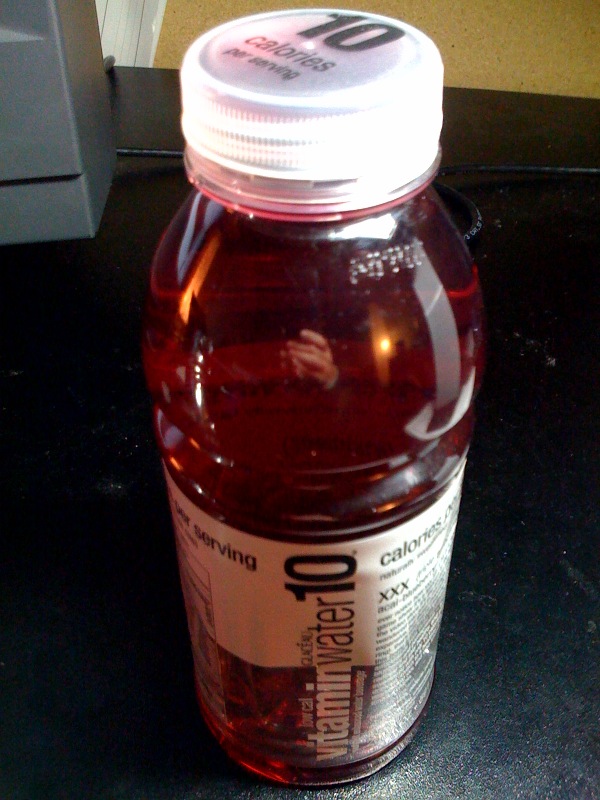Indoor color photograph, close-up of a cylindrical bottle of Vitamin Water sitting on a black, crumb-speckled countertop. The clear plastic bottle contains a see-through purplish-red liquid. Viewed from above, the bottle's opaque, round cap features black text reading "10 calories per serving." The label, which is white with black vertical text, prominently displays "vitamin water 10" and has partially legible calorie and ingredient information on either side, but the specifics are blurred.

Notably, there's a reflection in the upper portion of the bottle showing a person's hand holding a cell phone, likely the photographer. In the background to the left, a partial view of a gray or white appliance with a visible corner and cord is seen, along with a tan-colored object in the upper portion of the image.